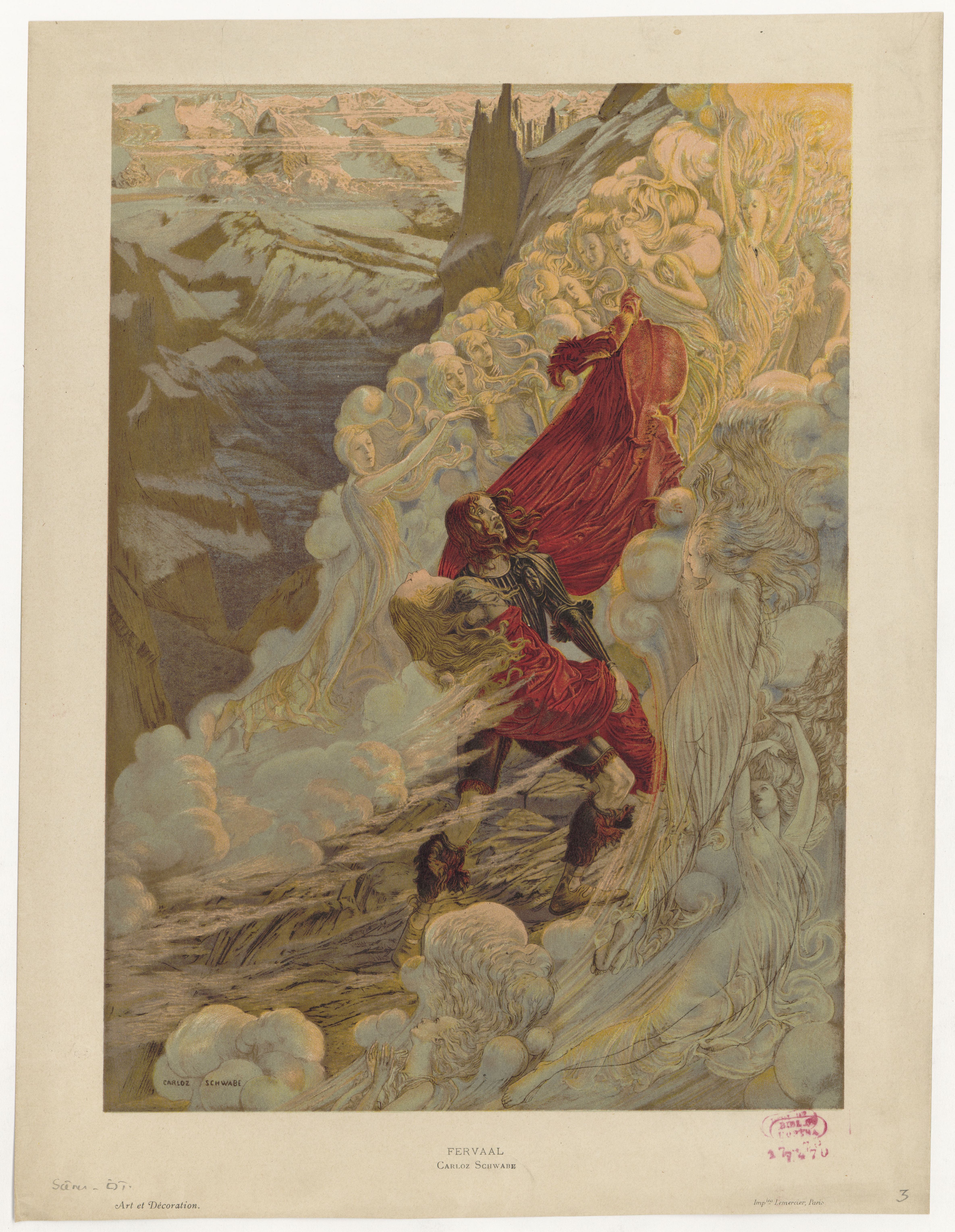A beautifully detailed painting on cream-colored canvas portrays a dramatic scene of ascension. Central to the image is a woman with amber-colored hair blowing forward, clad in an elaborate dark green and gold outfit. She is lifting another figure, a man draped in a flowing red blanket, presumably carrying him towards heaven. His head is tilted back, and his long hair clings to his back as one arm wraps around her neck and the other supports her knees.

Surrounding them on both sides are intricately drawn angelic figures, rendered in white, pointing upwards, guiding their ascent. The background features a landscape of gray, spiky mountains dusted with snow, adding to the painting’s ethereal atmosphere. A bright light emanates from the top right corner, bathing the scene in a divine glow, perhaps symbolizing heaven or a spiritual realm.

The painting is bordered by a one-inch cream margin and bears the text "Fravel" at the bottom, alongside an amber-colored stamp and the number three in the far bottom right corner. The artwork evokes a sense of timeless splendor, framed within the grandeur of old-fashioned artistry and steeped in warm tones.